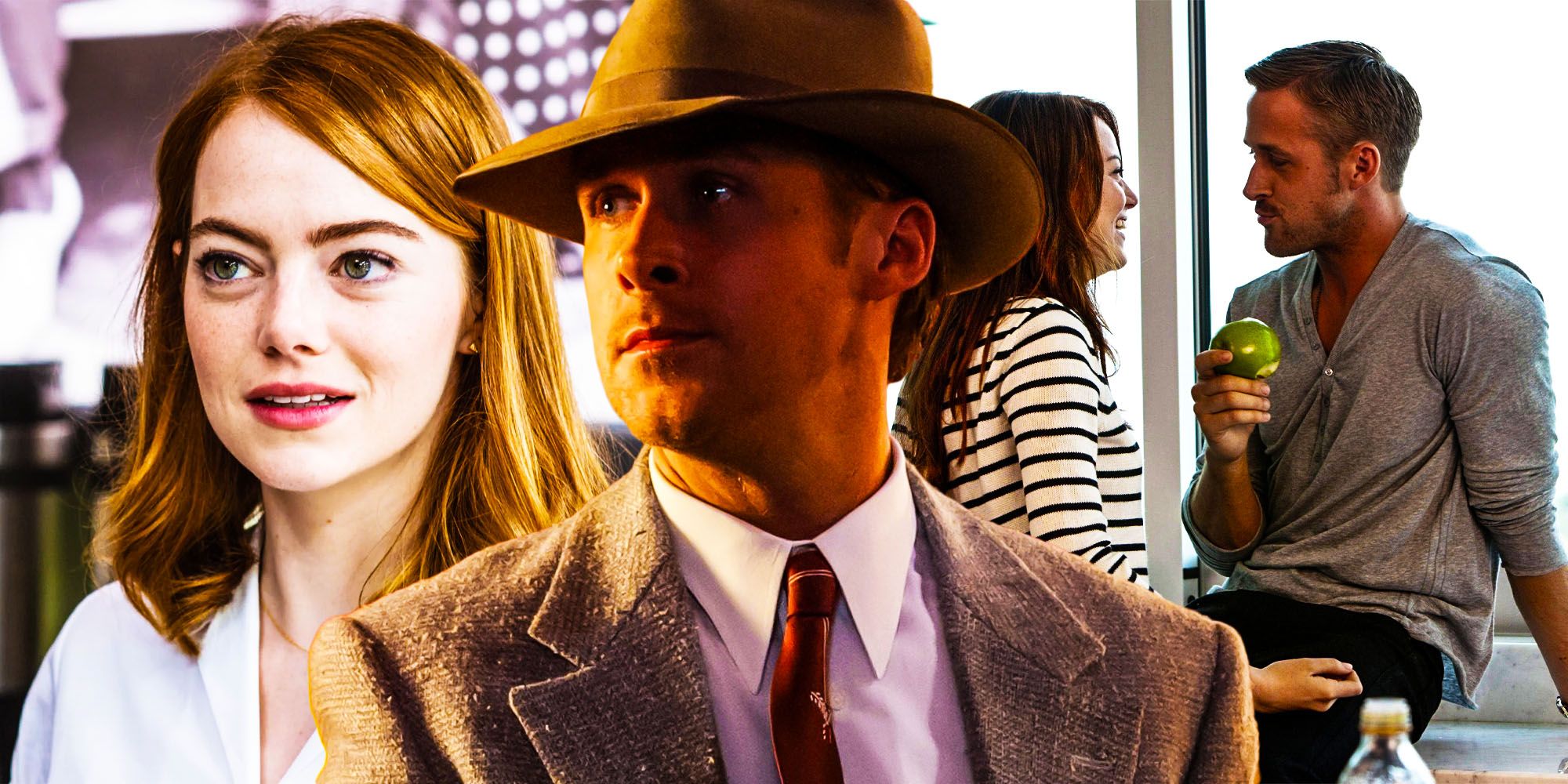In this image, which appears to be a movie poster or a scene from a film featuring lead actors Ryan Reynolds and Emma Watson, several details catch the eye. The background showcases a cozy room, complete with a large glass window. Near the window, Reynolds, dressed in a gray long-sleeved shirt rolled up to his elbows and black pants, is sitting on the windowsill. In his right hand, he holds a green apple with a few bites taken out of it, looking intently at Watson. Watson, in turn, stands near him, smiling warmly with her right hand resting on or near his left thigh. She is wearing a white shirt with horizontal black stripes and is looking back at Reynolds.

In the lower right corner of the image, the top of a water or soda bottle is visible, adding a casual detail to the scene. On the left side of the picture, there is another duo: Reynolds, this time wearing a tan suit with a white button-down shirt, a red tie, and an Indiana Jones-style hat, looking sideways. Behind him, Watson is visible again, sporting a white shirt and smiling while gazing sideways. Her long reddish hair is tucked behind her left ear, and she is wearing pink lipstick. The overlapping images and positions of the characters suggest a layered, perhaps complex narrative, emphasized by the multiple viewpoints and expressions captured in this single frame.